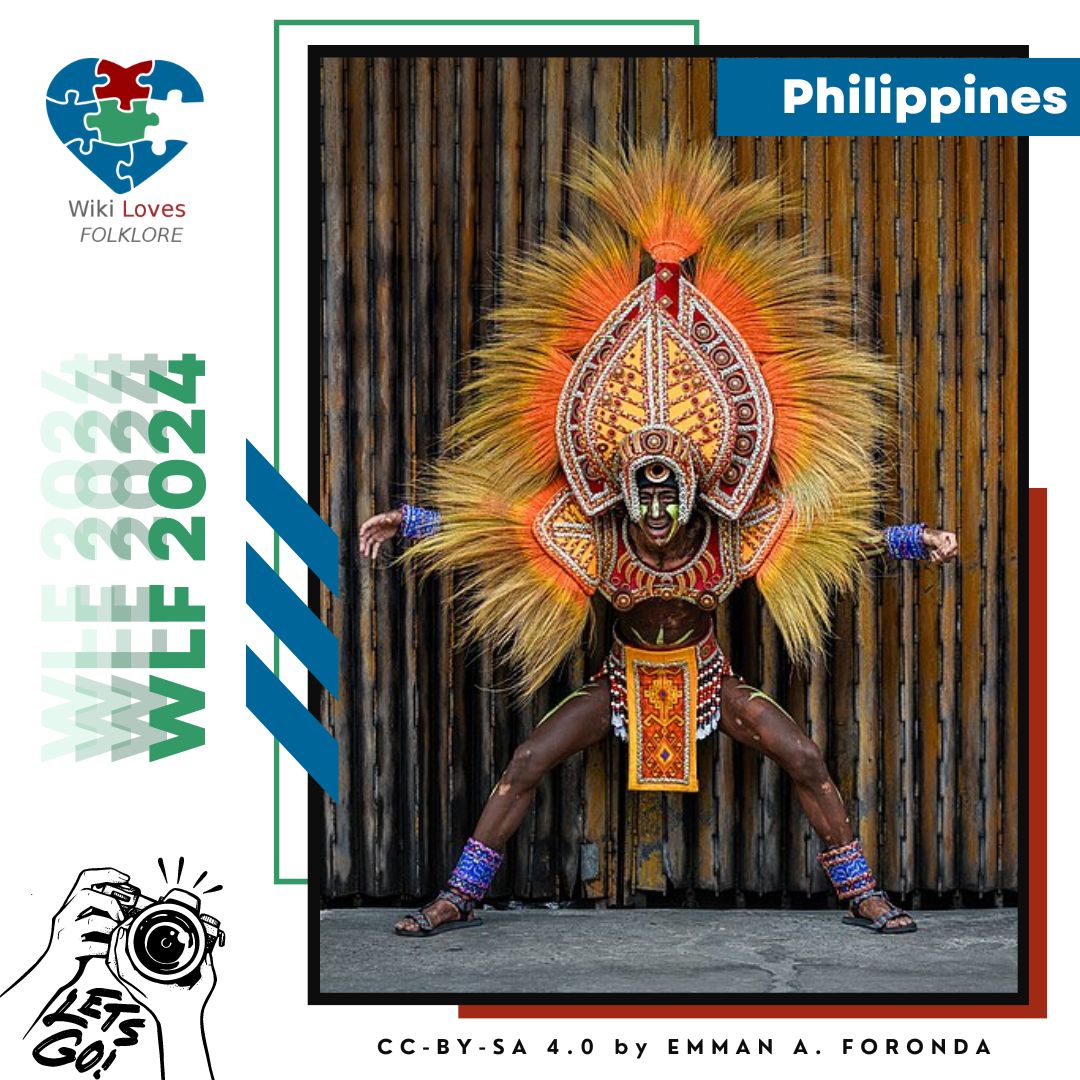The image is a vibrant promotional advertisement for Wiki Loves Folklore 2024, featuring the picturesque Philippines. Dominating the center, a man strikes a powerful warrior pose, legs astride and arms extended, dressed in traditional Filipino attire with an elaborate multicolored headdress adorned with orange and yellow grasses. His headdress and matching waist covering feature striking yellow, red, and white designs that spill into his breastplate and shoulders. White paint decorates his cheeks and nose, complementing his beaming smile. He stands against a rustic wooden background, sporting blue cuffs on his ankles and wrists, and sandals on his feet. The top left corner highlights the Wiki Loves Folklore heart logo made of puzzle pieces, while the bottom left corner displays clip art of someone holding a camera with the words "Let’s Go," inviting viewers to participate. The image caption credits read "CC by SA 4.0 by Emin A. Faranda."